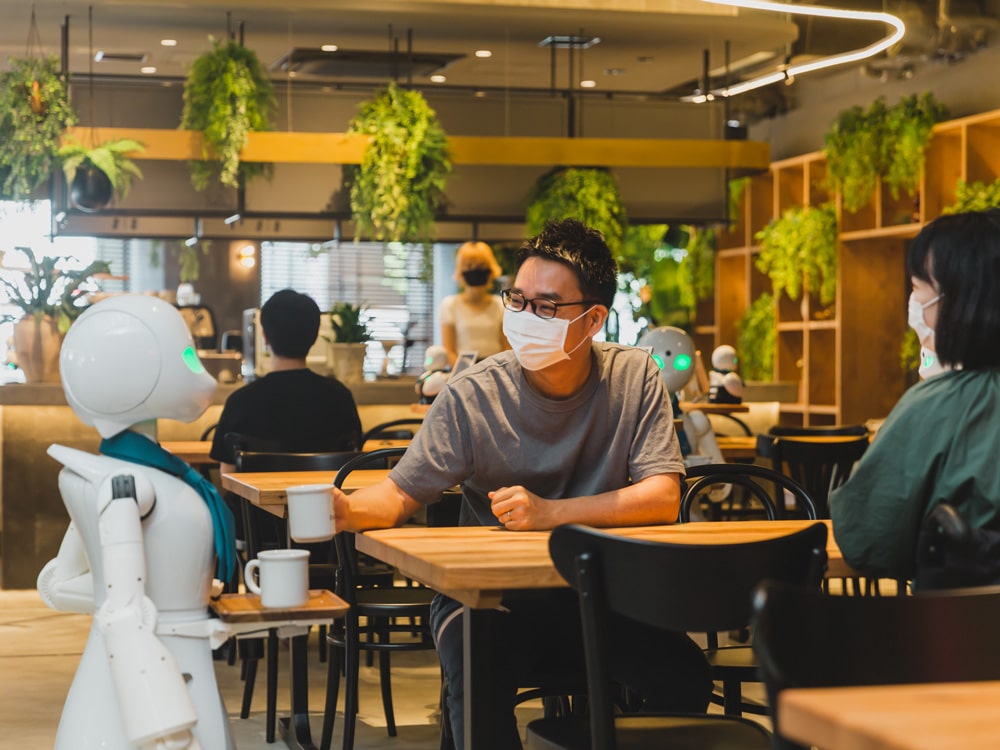In a bustling, greenery-filled cafe, a young Chinese couple, both wearing COVID masks, are seated at a whitewood table with black chairs. They are being served coffee by a small, white robot adorned with a blue scarf and featuring green glowing eyes. The man is reaching out to take a coffee cup from the robot's wooden tray. The background reveals more tables, additional patrons, another robot server, and lush green plants hanging from the ceiling on wooden shelves.